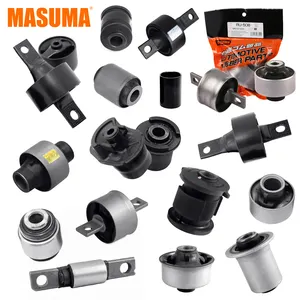The image prominently features a collection of metallic automotive parts from the brand "Masuma," which is displayed in bold, orange capital letters at the top left corner. The backdrop is a clean, white surface that accentuates the variety of mechanical components spread across it. These components, predominantly black and silver, are mostly cylindrical with various configurations; some have through-holes likely for bolts or rods, while others have flat bars intersecting their circular forms. There is a notable assortment of approximately 20 pieces, each differing slightly in size and design, yet all adhering to the common theme of automotive utility. In the top right corner, an orange and black package labeled "Automotive Spare Parts" is visible, suggesting these parts are prepackaged and ready for retail. The bag’s black top features a display hole for easy hanging, aligning with retail presentation standards. The components depicted appear to serve various functions within automotive systems, potentially including connections, casings, or other critical structural roles.